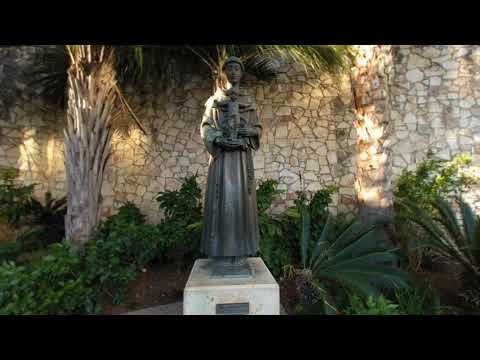This captivating outdoor photograph features a statue prominently centered within a lush garden. The horizontally-aligned, rectangular image is framed with thick black borders at the top and bottom, suggesting it might be a still from a video. The statue, a weathered gray figure possibly composed of concrete or metal like copper or brass, depicts a serene male saint or monk dressed in a long robe. He holds a smaller figure, perhaps a crucified Jesus or a baby, close to his midsection, the smaller figure's arms spread in a cross-like posture.

The statue stands on a square, white marble pedestal, adorned with an unreadable plaque. Surrounding the statue, the garden features a variety of green plants and bushes, thriving in brown earth. A palm tree trunk to the left extends its fronds overhead, and a sturdy, tall white stone wall dappled with sunlight forms a backdrop, enhancing the tranquil garden scene.